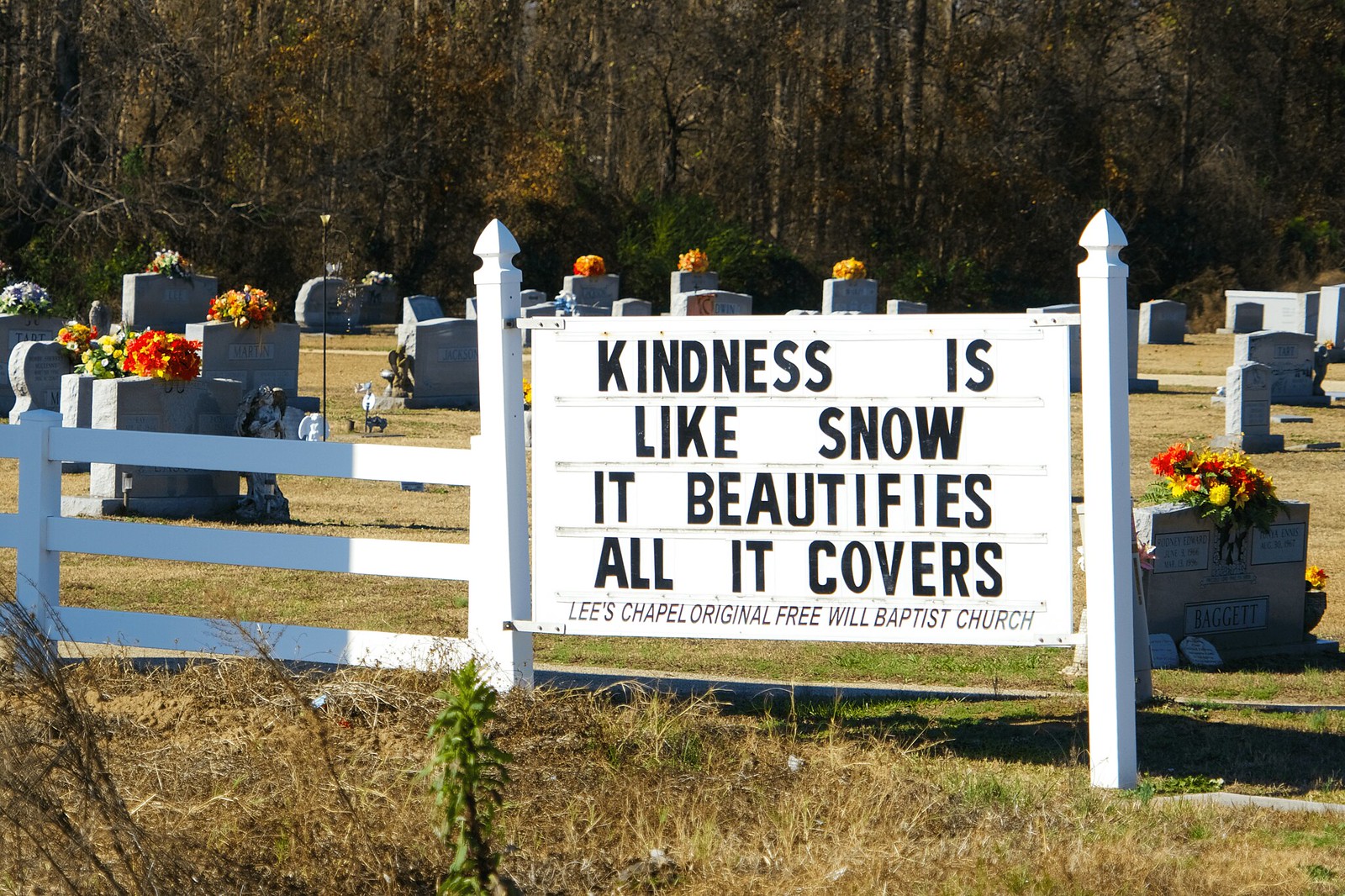A bright, sunlit photograph captures an old-time cemetery on a clear day. The scene is enclosed by a white wooden fence, to which a prominent white sign is affixed. The sign bears the inscription, "Kindness is like snow; it beautifies all it covers," and below that, "Lee's Chapel Original Free Will Baptist Church." Within the fenced area, aged headstones, broad and seemingly made of concrete, stand solemnly, many adorned with bouquets of flowers. The grass around the headstones is neatly mowed, adding to the serene atmosphere. In the background, a dense woodland provides a natural, tranquil backdrop to the historic resting place.